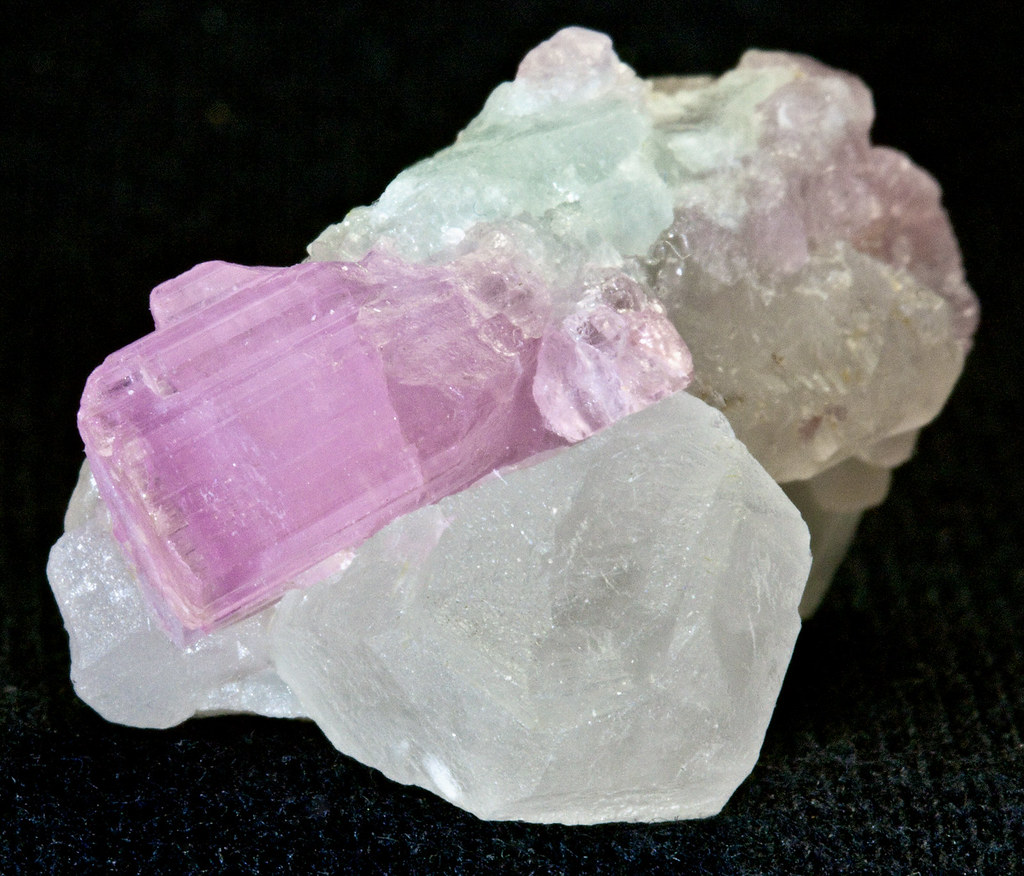This is an extremely close-up image of a multifaceted crystal, captured with such detail that it appears to be taken from a professional website. The crystal dominates the frame, set against a predominantly black background. The top left and right corners are solid black, while the lower section of the background features subtle specks of white, blue, and yellow, suggesting it might be resting on a multicolored surface.

The crystal itself is a mesmerizing blend of shapes and colors. It has a rounded front with a prominent rectangular section that is a vibrant, brilliant pink, fading into a lighter pink at one corner. This striking pink area sits atop a larger, white crystal base. Above the pink, there is a delicate sea glass blue segment that adds to the crystal's charm. On the right-hand side, hues of beige and light pink intermix, contributing to its intricate coloration. Despite being a single piece, the crystal's diverse color palette and shapes create an illusion of multiple segments seamlessly fused together.